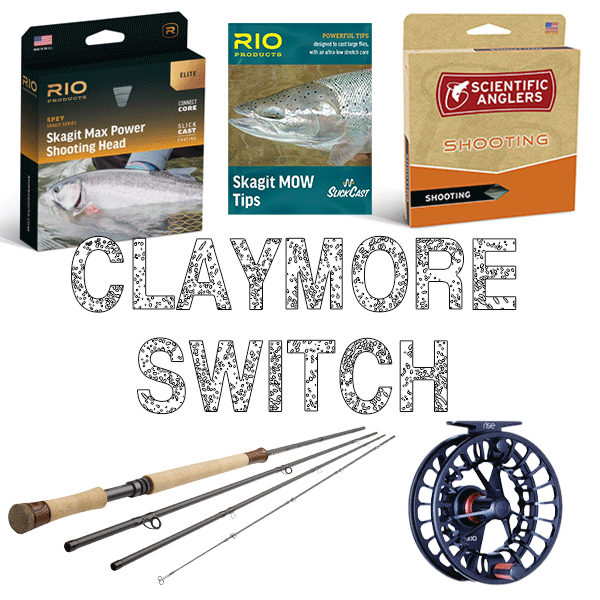This advertisement for fly fishing lures is set against a transparent background and prominently features three distinct accessory boxes at the top. The leftmost box, labeled "Rio Skagit Maxx Power Shooting Head," is a small black square with an image of a large silver fish. The middle box is teal and reads "Skagit Moe Tips," also showcasing a silver fish with black dots. The rightmost box has a cardboard-colored base with an orange border, featuring the Scientific Anglers logo and the word "Shooting" in red and white text. Each box represents a different Rio or Scientific Anglers product.

Centered in the advertisement, the text "Claymore Switch" is displayed in large white letters with black outlines and black dots, likely indicating the name of the fly fishing rod featured below. To the bottom left, the rod is shown in several pieces, characterized by its black segments and tan handle. On the bottom right, there is a black metal reel, visually similar to an open metal hubcap, completing the fishing setup.

This detailed and color-rich composition emphasizes the variety and quality of the fly fishing accessories offered, making it a comprehensive and eye-catching advertisement for any fishing enthusiast.